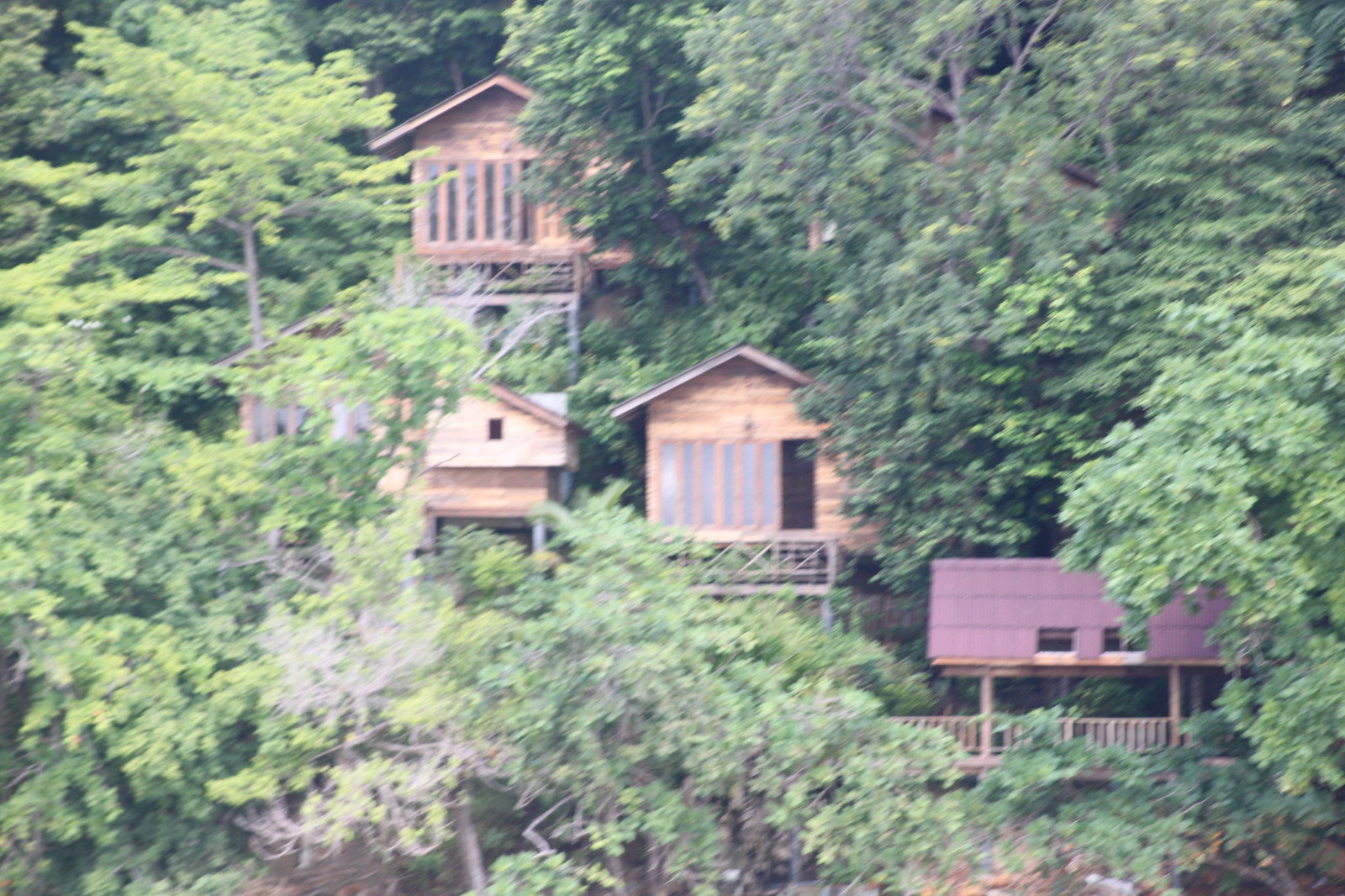The photograph captures a densely wooded jungle or forest scene illuminated by daylight streaming from the left, creating a play of mid-tone greens, lime-like yellows, and darker drooping foliage on the right. Nestled among the thick greenery are multiple wooden huts and cabins, built on stilts and featuring a variety of architectural details. Some structures have glass fronts or multi-paneled windows, while others display simple cutouts for windows. One prominent cabin in the bottom right corner showcases horizontal wooden panel fencing, topped by what appears to be a roof-covered patio. Just above and slightly obscured by the foliage, other wooden structures stack vertically, indicating a complex, multi-level arrangement of these treehouse-style homes. Despite some elements being blurred, the image clearly reveals a harmonious blend of man-made dwellings with the surrounding natural environment, creating a serene and intricate living space ensconced within the dense greenery.